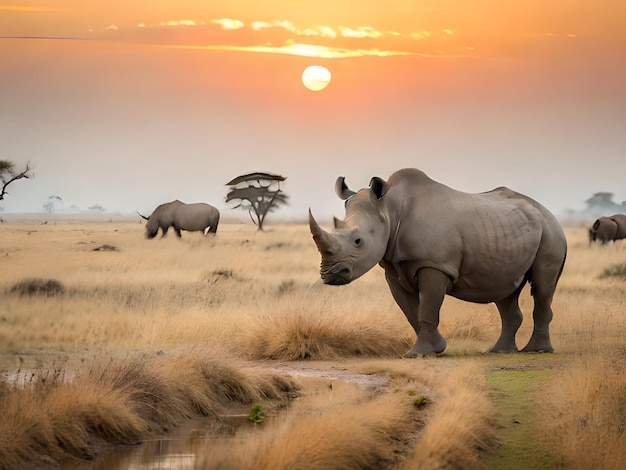The photograph captures a vivid nature scene set on the African plains, highlighting a trio of rhinoceroses amidst a backdrop of tall, golden-brown grass interspersed with patches of green. The central focus is a solid gray rhinoceros positioned slightly off-center to the right, gazing leftward with its prominent single horn, erect ears, and a small black eye. Further back, another rhino's back end is barely visible on the right side and yet another rhino is grazing on the left. The landscape features sparse, barren trees and a small water patch in the bottom left corner. The sky is a breathtaking gradient of orange and light gray-blue, with a golden-yellow sun positioned in the top center, framed by feathery white clouds.